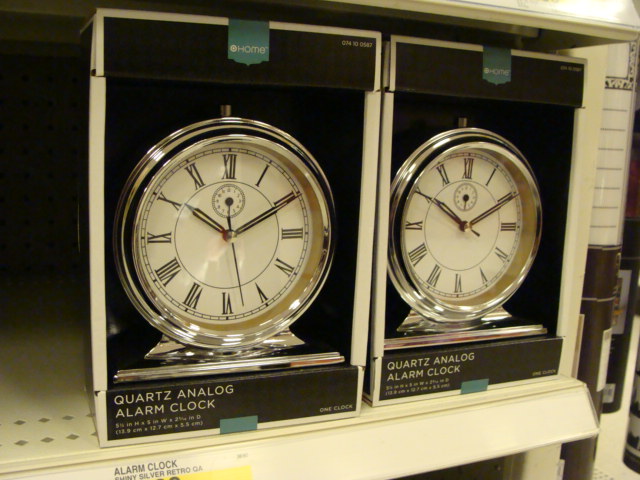This photograph captures a display of two identical silver alarm clocks on a store shelf, neatly arranged in their original packaging. The packaging is sleek and modern, featuring a black background with a white border and a teal-colored logo. Prominently displayed at the top center of each box is the word "Home." The alarm clocks themselves are circular in shape and rest on short square pedestals, adding a touch of elegance to their design. The clock faces are white, adorned with black Roman numerals, and feature a smaller sub-dial just below the number 12. The hands of the clock, including the hour, minute, and second hands, are elegantly designed with cut-out outlines. While both clocks are identical and encased in the same packaging, each one displays a different time, hinting at their functionality. The price tag is out of frame, though a label reading "alarm clock" is visible.